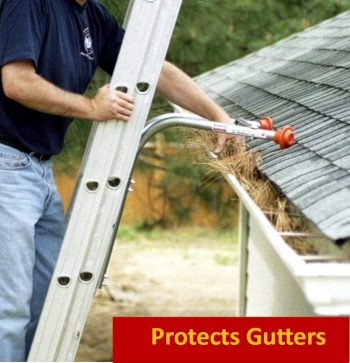This is an outdoor product listing image depicting a man cleaning the gutters of his house while demonstrating the use of "ladder horns" to protect the gutters. The photo is vertically rectangular and primarily focuses on the man, who is dressed in a navy blue short sleeve shirt and light blue jeans. The man, a white male, is standing on the rungs of an extension ladder made of light gray metal, holding the side of the ladder with his right hand while using his left hand to remove brown grass clippings and debris from a white gutter. The ladder is equipped with "ladder horns" that extend from the ladder, preventing it from resting directly on the gutters. The blurry background at the top of the image shows green leafy trees. The rooftop on the right side of the image features slanted shingles in white to light gray. At the bottom right corner, a red rectangular background displays the text "Protects Gutters" in yellow capital letters, emphasizing the product's benefit.